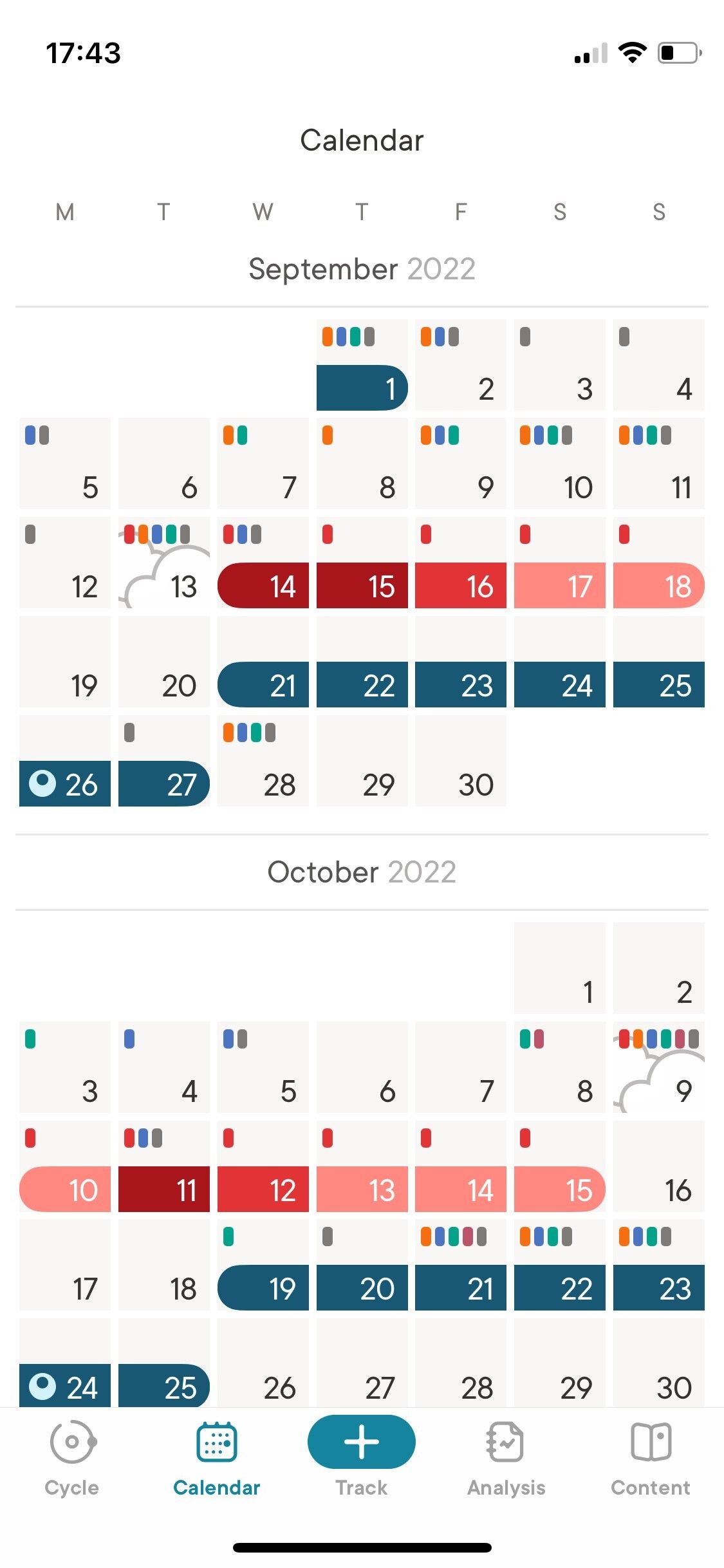A screenshot of a smartphone calendar app, displayed on a white background, reveals an organized yet busy schedule. The phone shows a military time of 17:43 (5:43 PM) in the top right corner, accompanied by two bars of signal strength and a battery indicator that's at approximately 33%. Below the status bar, the word "Calendar" is written in black, narrow font.

The main content shows the months of September and October 2022. "September" is in bold black text, while "2022" appears in gray. Various dates are highlighted with colored dots - orange, blue, green, purple, and additionally red - to indicate multiple events occurring on the same day. The 13th of September is exceptionally busy, showcasing five different color-coded engagements. Some dates are blank, signifying no scheduled activities.

Directly below the September calendar is the October 2022 calendar, which introduces a sixth color to the scheme. Again, multiple dates are marked with a combination of the colors, illustrating diverse activities. A cloud icon appears over particularly busy days, perhaps indicating poor weather or another contextual detail.

This detailed visual representation likely helps the user track and manage their multifaceted schedule effectively, despite the dense visual information suggesting a high level of activity or complexity in their plans.